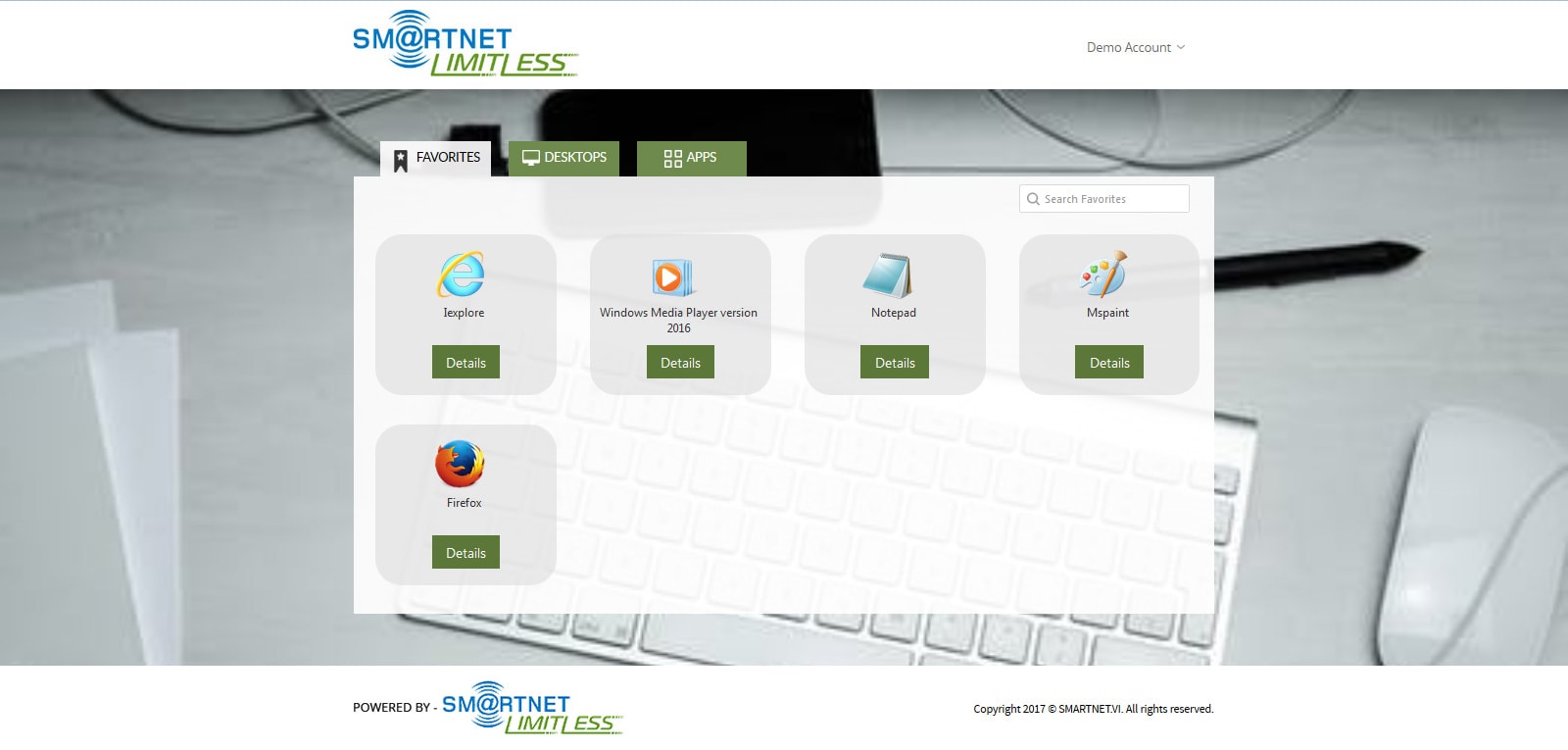The image depicts a clean, modern desktop interface from a platform called "Smart Net Limitless." The background is a pristine, white digital workspace that gives a faux woodgrain appearance, and features a white wireless mouse and keyboard with a few documents neatly placed to the left.

At the top of the interface, the "Smart Net" logo is presented in a stylized font with a unique 'a' character that resembles the '@' symbol. Soundwave-like curves emanate from the 'a,' giving it a dynamic, tech-savvy look. Immediately below, the word "Limitless" is displayed in bold, fully-spelled-out letters, indented to the right.

A dropdown menu labeled "Demo Account" allows users to select different options. Beneath this is a white dialog box where various software options are listed under the "Favorites" section. These include:

- **Internet Explorer**: Represented by its classic blue icon, with a green button for additional details below.
- **Windows Media Player**: Represented by the 2016 version icon, also accompanied by a details button.
- **Notepad**: Indicated by a blue notepad icon, again with a details section underneath.
- **MS Paint**: Listed in this section as well.
- **Firefox**: Appearing in the subsequent row.

To the lower left of the interface, in a smaller font, it reads "Powered by Smart Net Limitless." The copyright information is demurely placed underneath this logo. 

Overall, the image exudes a polished, professional feel suitable for a tech-savvy audience.